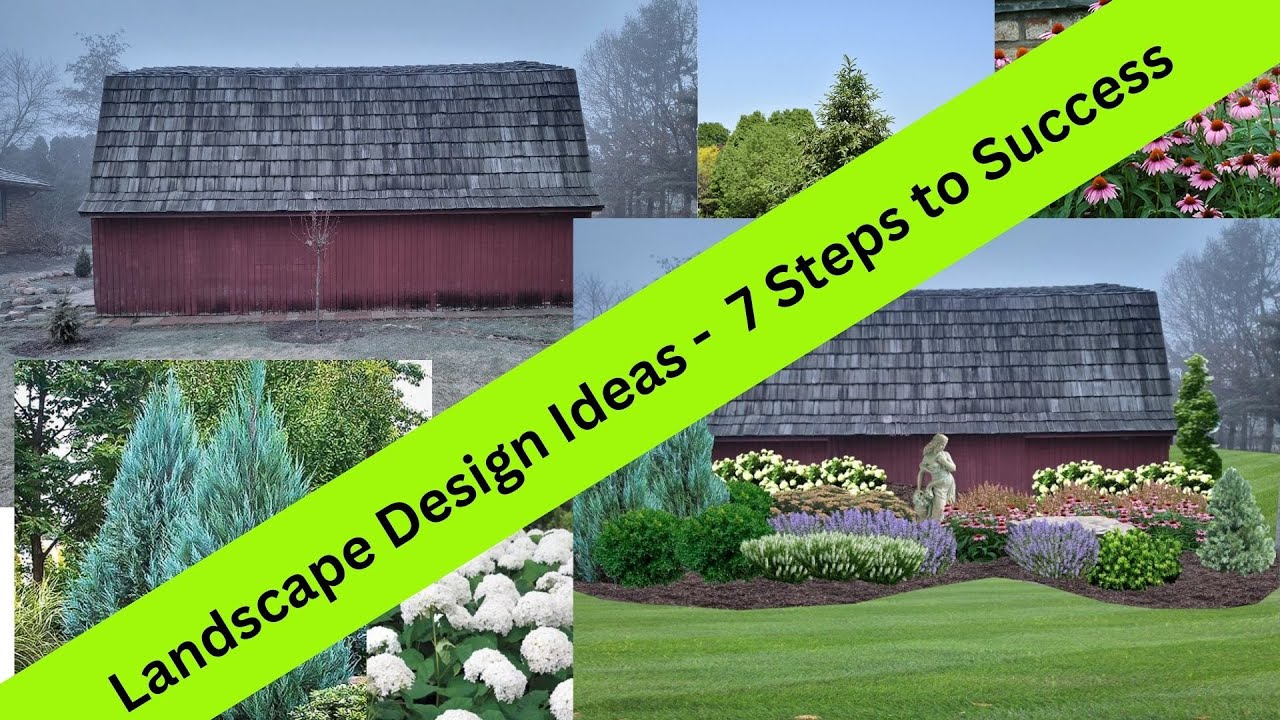The image showcases "Landscape Design Ideas: Seven Steps to Success" in black font on a bright neon green ribbon that spans diagonally from the lower left to the upper right. This visually appealing collage comprises five different images highlighting various aspects of landscape design. In the top left corner, there's a maroon barn with a dark charcoal gray rooftop, surrounded by dirt and two bushes, enveloped by a dull bluish sky. The bottom right segment reveals a meticulously designed landscape featuring freshly cut grass, well-maintained flower beds with lavender, white, and pink flowers, and a statue amid lush greenery. Other sections illustrate a foggy backdrop with sunlight piercing through, showcasing trees and additional plants. The entire composition is landscape-oriented, reflecting diverse stages and elements of successful landscape design through vibrant colors like green, maroon, pink, purple, and blue.